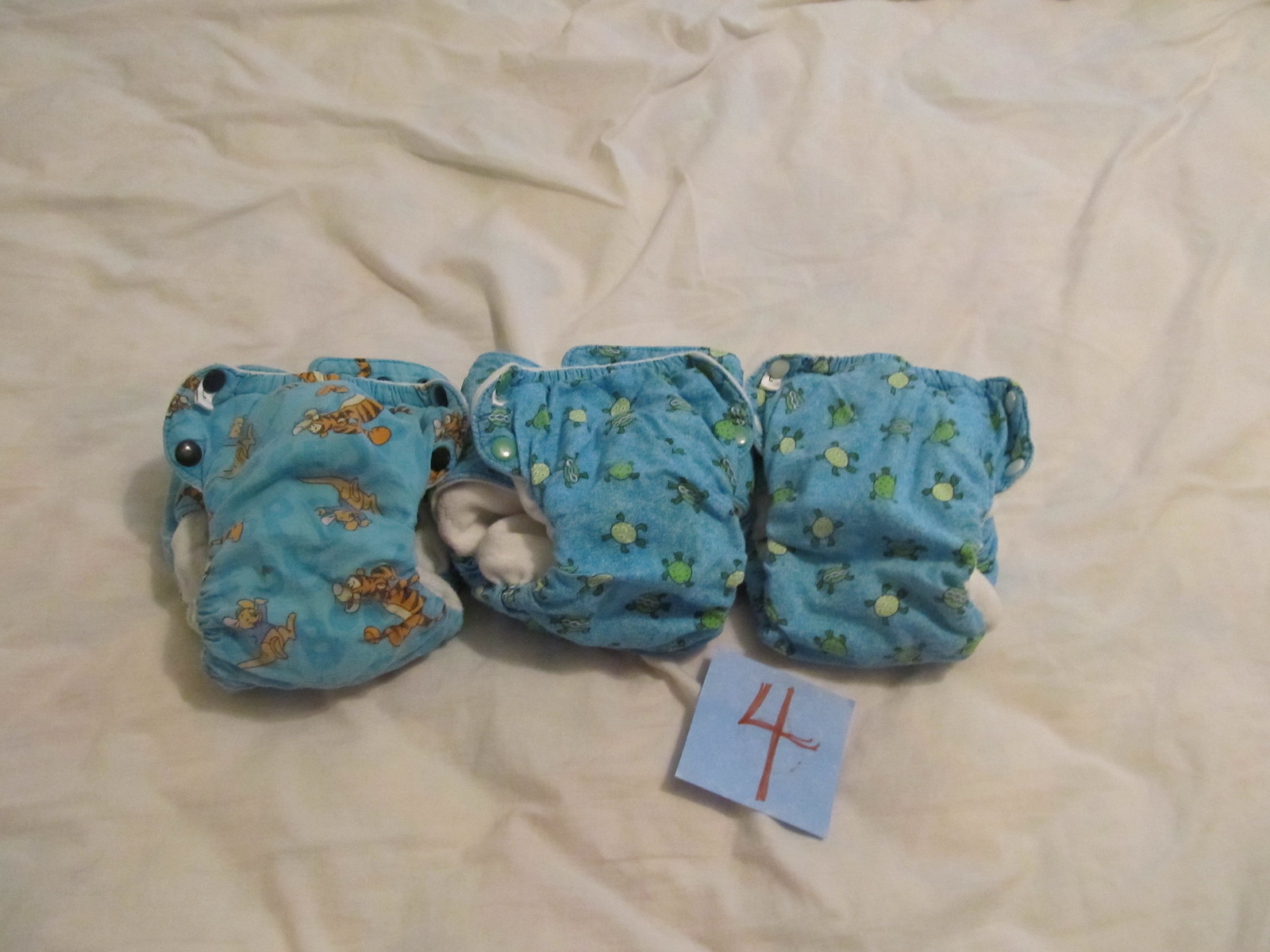In this dimly lit, slightly out-of-focus indoor color photograph, three blue diaper covers are neatly arranged side by side on a wrinkled, off-white cotton sheet. These covers, which are used for cloth diapers or to dress up disposable ones, feature snaps or buttons on the sides for securing them around a baby's waist. 

The left-most diaper cover is adorned with black buttons and vibrant Disney characters, specifically Tigger and Rue from Winnie the Pooh. Peeking out from this cover, white bunches of cloth suggest the presence of a cloth diaper inside. Both the center and right diaper covers share the same light blue color and are decorated with sea turtle patterns. 

Below the center and right diaper covers, a light blue square piece of paper (resembling a post-it note) is visible, bearing the number "4" written in red crayon or marker, indicating perhaps an order or a category. The overall ambiance of the photograph conveys a sense of gentle, practical care, emphasized by the soft, cottony backdrop and the slightly used appearance of the items.